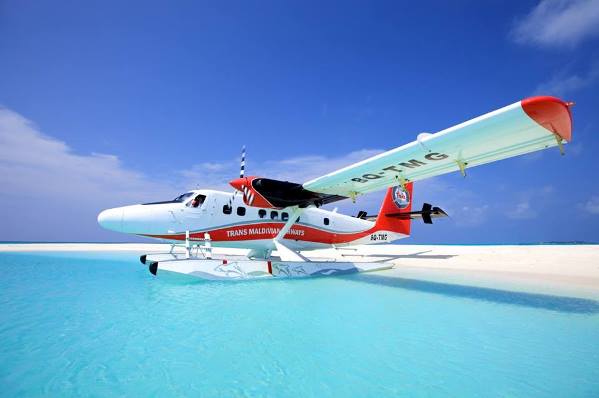This detailed image features a small white seaplane with distinctive red details floating on extraordinarily clear, vibrant blue water. The aircraft, equipped with two engines mounted on either side of its wings, has a red banner below its body that partially reads "Trans...", indicating its operator, possibly Trans Maldovia. The plane's wing tips are also red, and on the underside of one wing, the registration "BQ-TMG" is visible in bold black letters. The airplane, which has six small square windows down its side and appears to seat six rows of passengers, rests gracefully on its pontoon floats. In the backdrop, the blue sky is punctuated by scattered white clouds, enhancing the idyllic setting. There's a strip of light white sand visible behind the plane, adding to the sense of an isolated, serene island environment. The scene is captured outdoors with the seaplane slightly angled diagonally, perfectly centered in the frame against the picturesque sky, water, and sand.